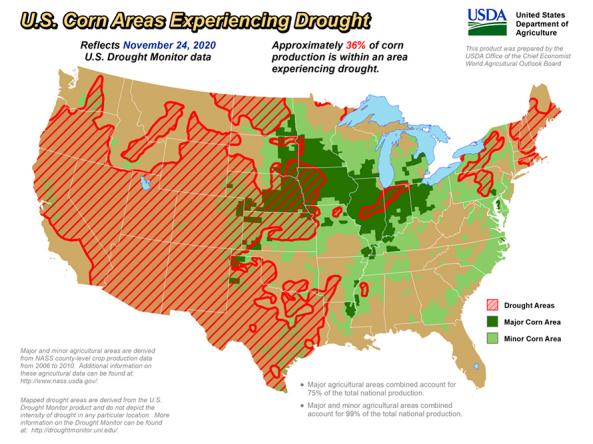This detailed map of the continental United States from the USDA Office of the Chief Economist Wheat Agricultural Outlook Board highlights regions affected by drought using data from the U.S. Drought Monitor as of November 24, 2020. Approximately 36% of the country’s corn production is within areas experiencing drought. The map employs a color-coded legend: red areas with diagonal lines represent drought-impacted regions, concentrated primarily in the West and Midwest; dark green areas indicate major corn production zones, predominantly in the Midwest; and light green areas mark minor corn production zones, mostly situated along the East Coast. The text on the map specifies that the major and minor agricultural areas are based on NASS county-level crop production data from 2006 to 2010, and outlines that these combined areas account for 99% of the total national production. The map’s layout features no border and uses a landscape rectangular format with a white background. The title "U.S. Corn Areas Experiencing Drought" is displayed in yellow font with a black shadow. Additional detailed information can be found in the four small font paragraphs below the map. Key entities and related information are signposted by the USDA and the U.S. Drought Monitor websites for further insights into the drought conditions and agricultural impact.